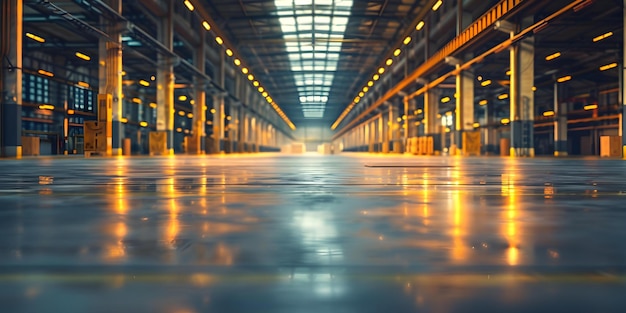This image captures the eerie, liminal atmosphere of what appears to be an abandoned industrial structure. The perspective is from a low angle, almost as if the camera was placed on the wet, reflective concrete floor, looking down a long, narrow corridor. The facility could be a deserted warehouse, train station, or parking garage, given the array of potential indicators like yellow stanchions, concrete block columns with blue and yellow stripes, and potential train alleyways. The ceiling, presumably all glass, hints at a single-story facility, though it could have offices above certain areas. Numerous yellow-orange lights line the extensive hallway, casting their glow onto the floor and accentuating the orange-yellow-gray tones that dominate the scene. The overall emptiness, with no people or identifying features, enhances the liminal quality of this industrial, metal, and concrete landscape.